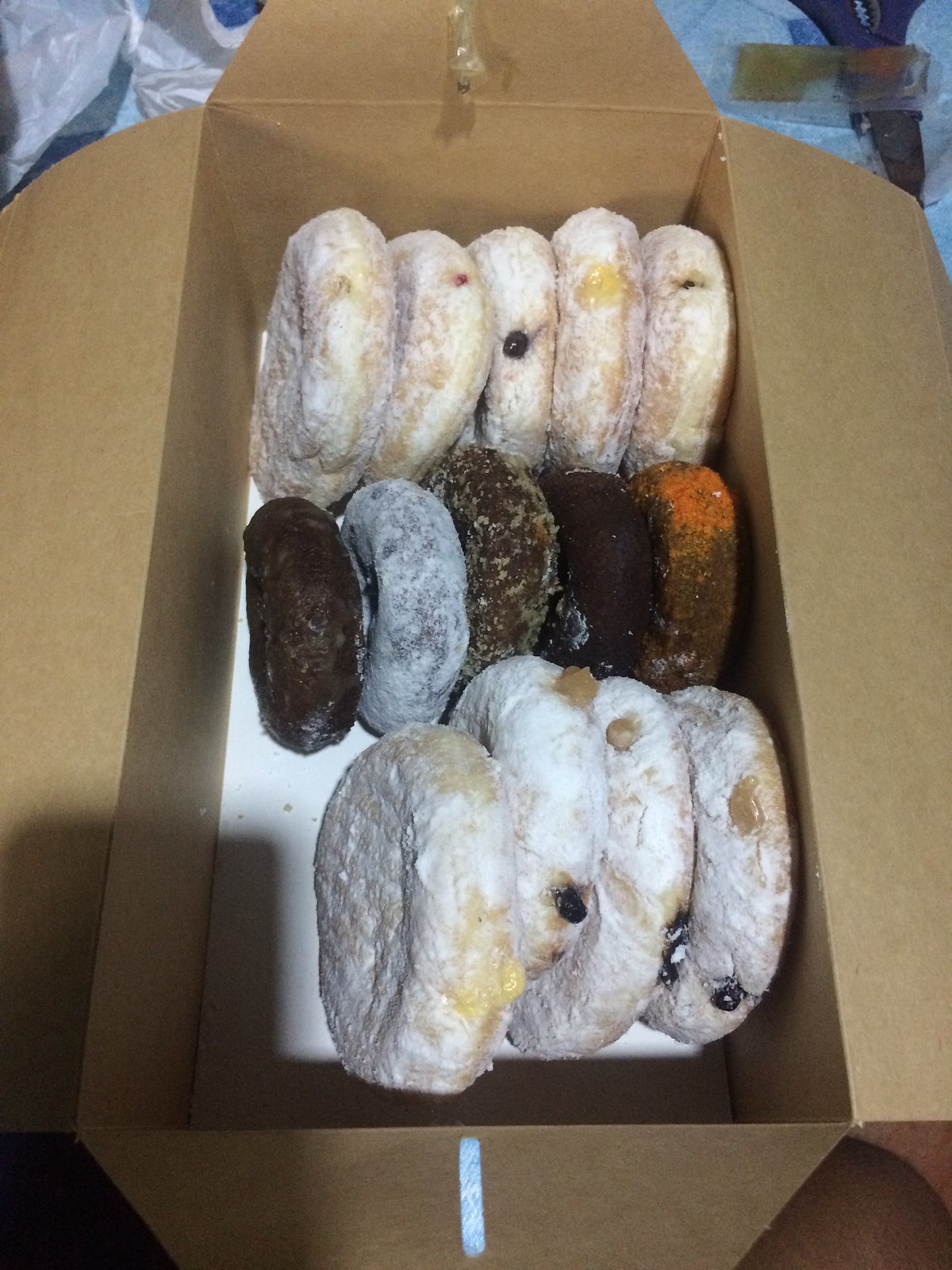The image features an open rectangular brown cardboard takeaway box containing an assortment of 14 circular donuts, meticulously arranged in rows. The top row showcases five donuts covered in white powdered sugar, each embedded with dark circular fruits, possibly raisins or blueberries. Below them, the middle row contains five chocolate donuts, differentiated by their variations: some are purely glazed chocolate, one has a dusting of white powder, and others appear to be cake donuts, with one exhibiting a light brown hue and a hint of orange, likely from carrot powder. The final row mirrors the top row with four more powdered donuts, similarly studded with dark fruits. The box is lined with a white sheet of paper to prevent the donuts from falling through. In the background, partially visible, are a pair of scissors, a light-colored packet of sauce lying atop the scissors, and a peeking plastic bag, possibly the bag that originally contained the donuts.